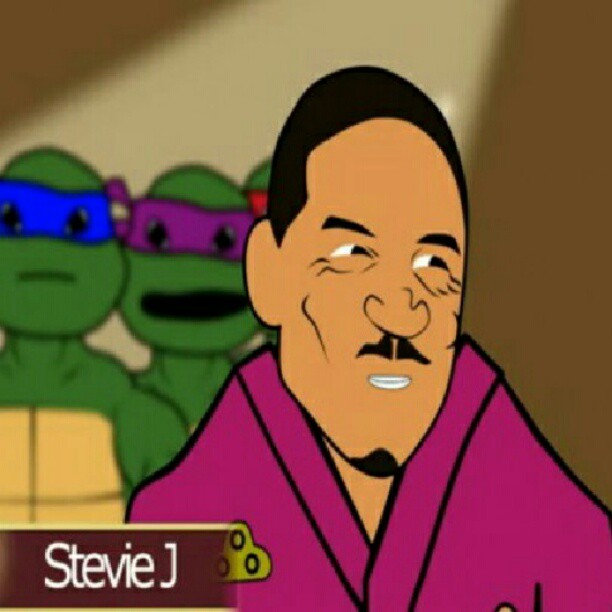The image appears to be a detailed cartoon illustration featuring a backdrop of crudely drawn Teenage Mutant Ninja Turtles. Leonardo, identifiable by his blue bandana, has a green complexion with a light brown undertone. Beside him is Donatello, distinguished by his purple headband, with only his head visible. To Donatello's right is Raphael, identifiable by his red bandana, partially obscured by the central figure in the image.

At the forefront stands a cartoonishly depicted African American man with a small mustache, a goatee under his chin, and an angry expression. He wears a purple robe adorned with an emblem that resembles brass knuckles on the right side. His eyes are squinted, and he has a shifty, sidelong gaze. The man’s slightly shifty demeanor is accentuated by a TV smile.

In the bottom left corner of the image, there is a dark gray band with the text "Stevie J." displayed in white letters.